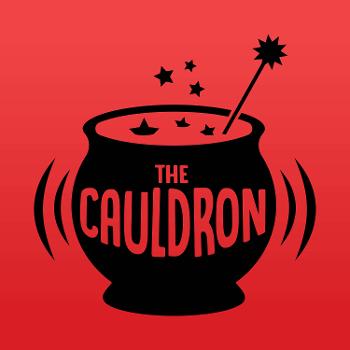The image features a bright red background and a central stylized black cauldron, evoking a business logo or brand image. The cauldron's simplistic silhouette includes the text "THE CAULDRON" in black capital letters stretching across its width. There are action lines resembling parentheses on either side of the cauldron, creating an animated effect as if it's shaking or boiling. Instead of steam or bubbles, black stars emerge from the top, with some stars also submerged in the red liquid within the cauldron, blending seamlessly with the background. Protruding from the cauldron towards the upper right is a stick or wand, adorned with an intricately detailed spiky nine-point black star at its tip. The overall design combines elements of magical imagery with a minimalist aesthetic.